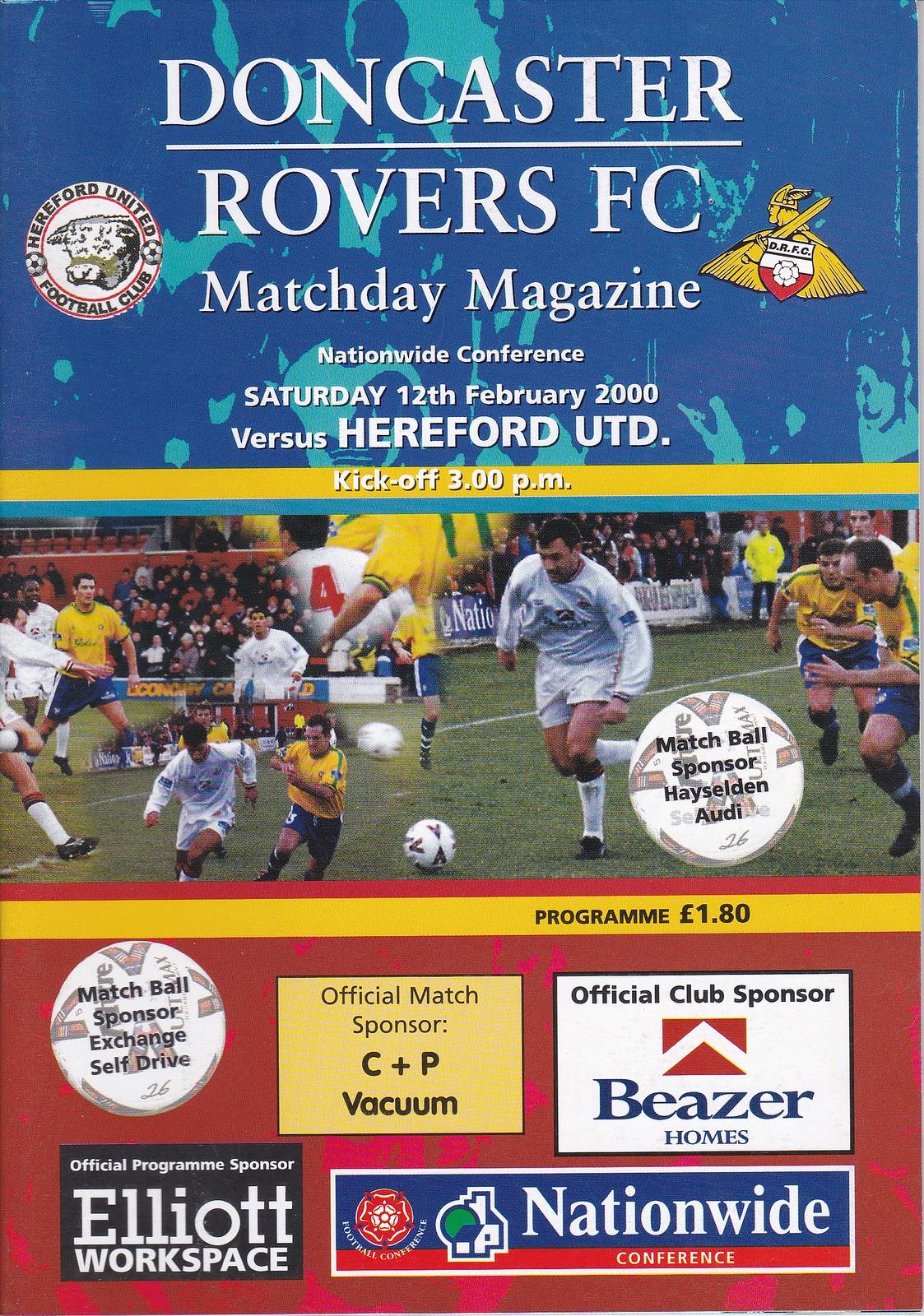This detailed magazine cover for the game program between Doncaster Rovers and Hereford United is arranged in three distinct sections. The upper third boasts a blue and teal graffiti-styled background, featuring prominently in bold, uppercase white font, "DONCASTER ROVERS FC." Flanking this text are the logos of both teams: on the left, an emblem of Hereford United Football Club depicting a small cow within a circle, and on the right, a golden side-view of a Viking with a shield. Below this, the title "Match Day Magazine" is displayed, followed by "Nationwide Conference," "Saturday, 12th February 2000," and "Versus Hereford UTD," all in capital letters. A yellow banner beneath this section announces the kickoff time at "3 p.m." 

The middle third of the cover features a dynamic collage of live-action shots from soccer matches, capturing players in motion—running, kicking, and vying for the ball. Prominent in this section is a white soccer ball with the text "Match Ball Sponsor Heyselden Audi" superimposed over it.

The lower third transitions into a red background with a horizontal gold stripe at the top, indicating in black print "Program £1.80." This section is replete with logos and sponsor information. On the left, another white circle with "Match Ball Sponsor Exchange Self-Drive" is present. To the right, a yellow square with "Official Match Sponsor C+P Vacuum" sits next to a white box labeled "Official Club Sponsor Beezer Homes." At the very bottom left, a black rectangle with white text reads "Official Program Sponsor Elliott Workspace," and a long horizontal rectangle with a blue top and red bottom denotes "Nationwide Conference."

Overall, this cover blends vibrant colors, team emblems, sponsor information, and action-packed imagery to convey the excitement and importance of the event.